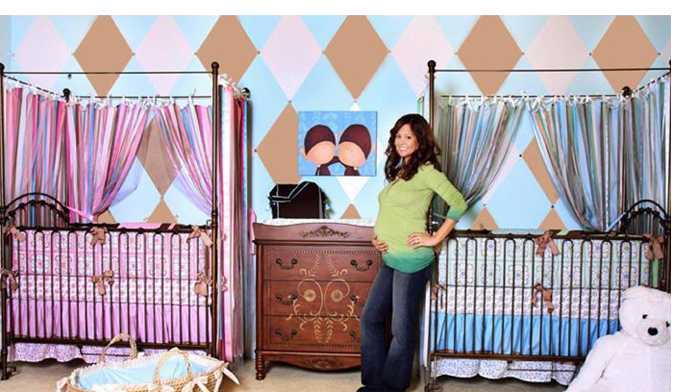In this color photograph, a visibly pregnant woman is standing in a nursery, seemingly designed for twins—a boy and a girl. She has long dark hair and is smiling at the camera, cradling her belly with her left hand while her right hand rests on her hip. She is dressed in a light green sweater that fades darker towards the bottom and wide-legged denim pants. The room's back wall features a whimsical pattern of pink, blue, and brown diamond shapes. To the left is a pink-themed crib draped with elegant curtains, accompanied by a woven Moses basket on the floor. On the right side, there is a matching crib in blue with similar curtained adornments. In the bottom right corner stands a plush white polar bear teddy bear. Centered between the cribs sits a wooden dresser with a gold pattern and a black bag on top, above which hangs a picture of two faceless baby heads. The serene and welcoming environment of the nursery is beautifully framed, reflecting thoughtful preparation for the arrival of twins.